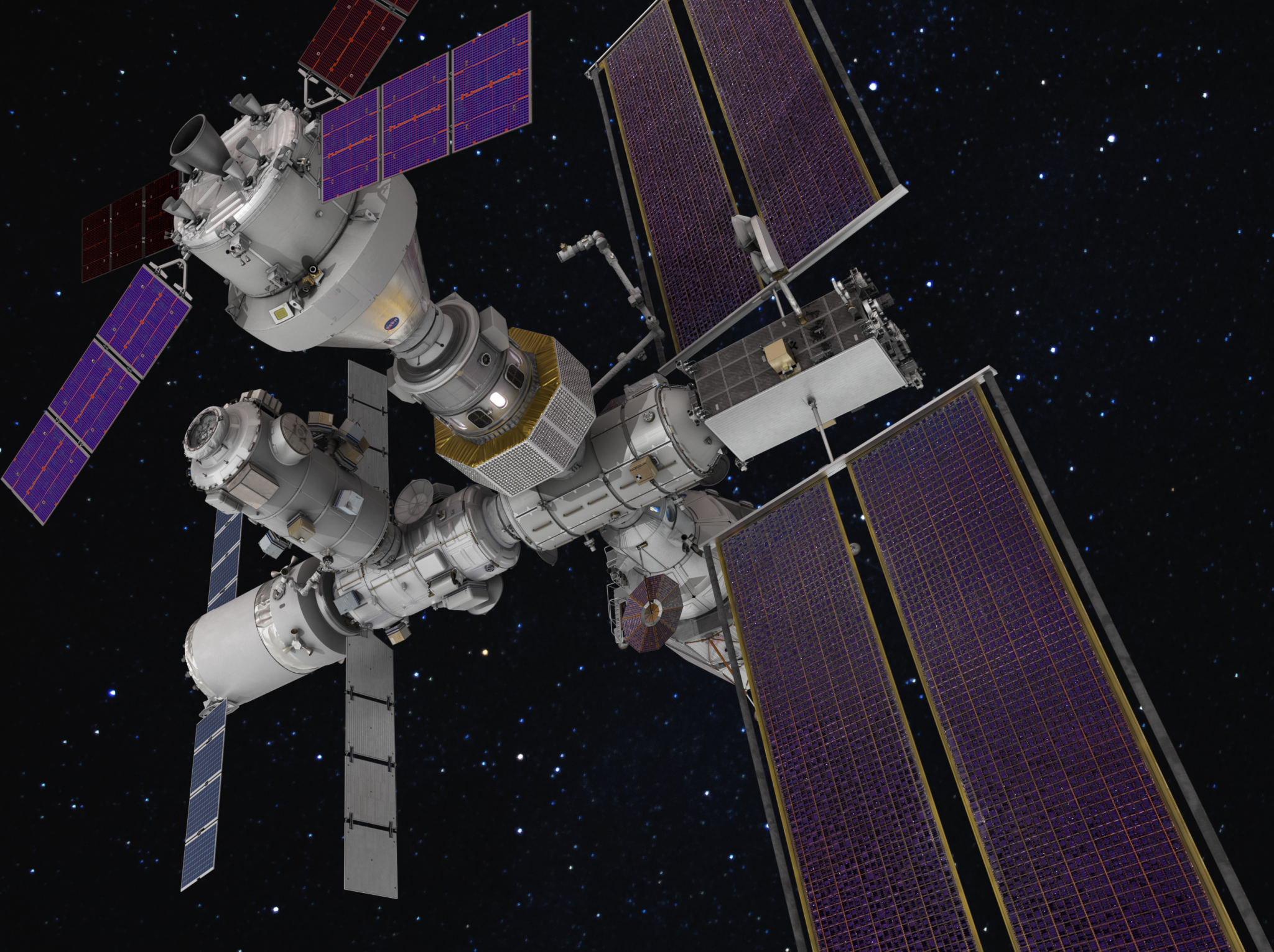The image is a detailed 3D rendering of the Gateway Space Station against a black sky sprinkled with blue, yellow, and white stars. The space station features various cylindrical segments, predominantly light gray to white, with notable parts adorned with glistening gold foil, probably for protection. The structure includes segments resembling escape pods and connecting corridors, giving a sense of a labyrinthine pathway. Surrounding these segments are multiple vibrant and eye-catching solar panels of varied shapes and sizes. The most striking are the bright royal purple solar panels, some rectangular, with two positioned in the lower half separated by a gap and others encircling cylindrical sections or extending perpendicularly with yellowing outlines. A cluster of smaller blue-hued panels can also be spotted. The scene is highly innovative, portraying a sophisticated and futuristic space habitat floating serenely amidst the celestial expanse.